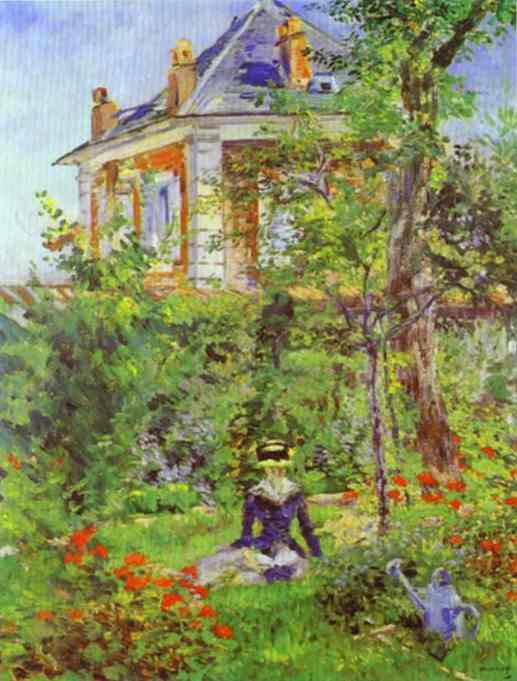In this vibrant impressionist painting, a woman is depicted seated or kneeling in a lush garden. She is situated on a grassy patch in the lower middle part of the artwork, dressed in a blue dress with a yellow and black hat. The focal point surrounding her includes an array of beautiful flowers—red and orange blooms—flourishing on either side and more in the foreground. A watering can is noticeably placed in front of her to her right.

The garden is depicted with vivid, loose brushstrokes, exuding life and energy. Towering to her right is a large tree, with various bushes brimming behind her. Further up in the background, the scene transitions into a slightly elevated hillside where a house stands prominently. This house, painted in vibrant red walls with white-framed windows, features a dark blue roof adorned with three chimney stacks—two on the left side and one facing us. The sky above is a striking gradient from bright blue at the top to lightening hues towards the horizon, creating an overall serene yet dynamic composition.